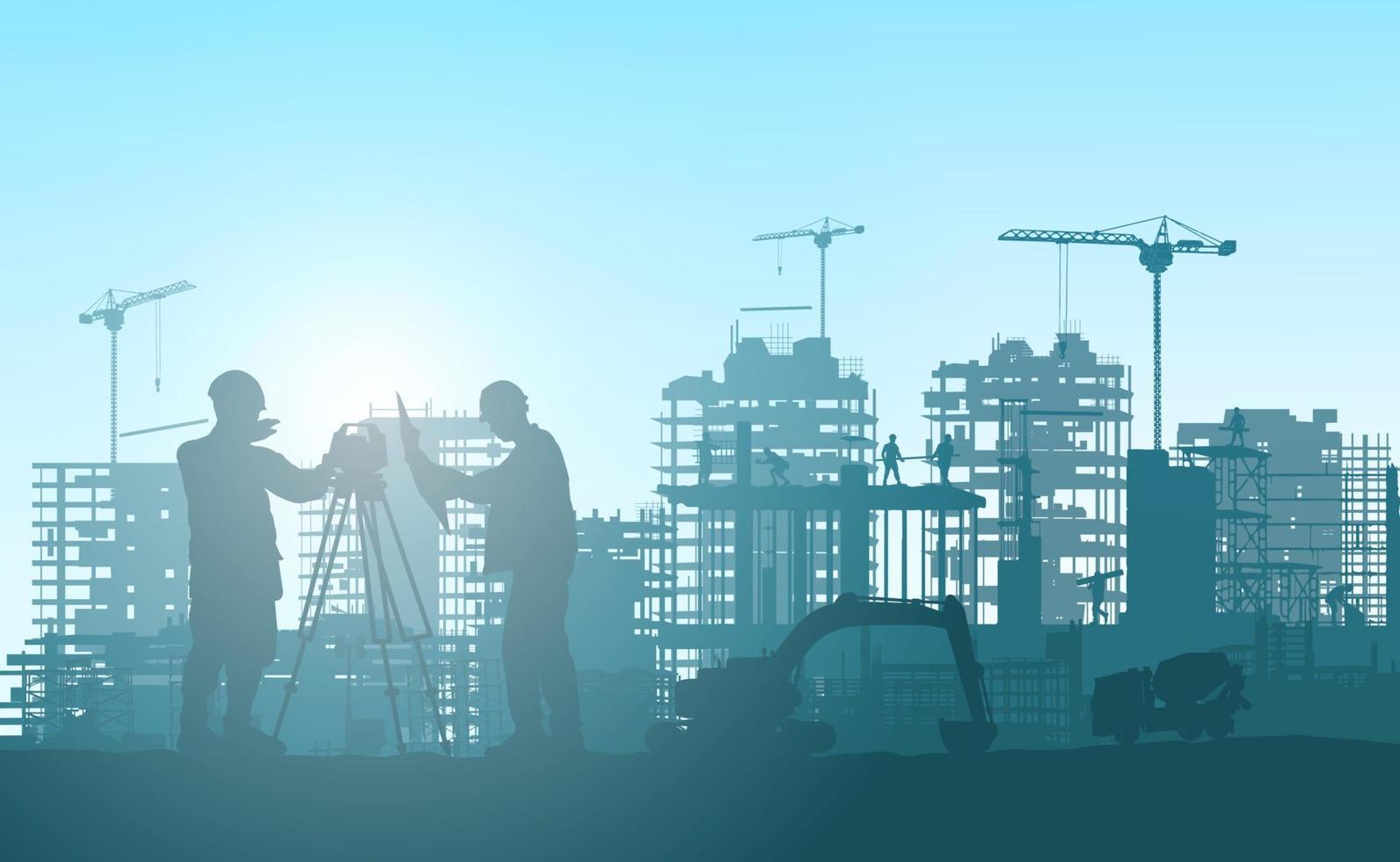The horizontally aligned rectangular image is a computer-generated vector illustration depicting a bustling construction site set against a city skyline. Dominating the lower part of the picture are five to six silhouetted buildings, stretching from left to right and showing the progress of urban development. In the foreground, on the far right, a cement truck and a backhoe loader stand facing each other, while on the left side, two construction workers are engaged in their tasks. The worker closest to the left appears to be a land surveyor, operating a laser device mounted on a tripod. Adjacent to him, another worker holds what might be blueprints or a map. Both workers, along with their equipment, are silhouetted in dark gray or black.

Above this busy scene, the sky is a gradient of light blue, with the area towards the left displaying a whitish tinge, suggestive of the sun's position. Towering cranes are strategically placed across the skyline—one on the far left, one in the middle, and one on the right—indicating ongoing high-rise construction. Scaffolding is visible on several buildings, highlighting the active nature of the construction. The overall image is rich in detail yet rendered with silhouettes, emphasizing the dynamic and industrious ambiance of the evolving city.